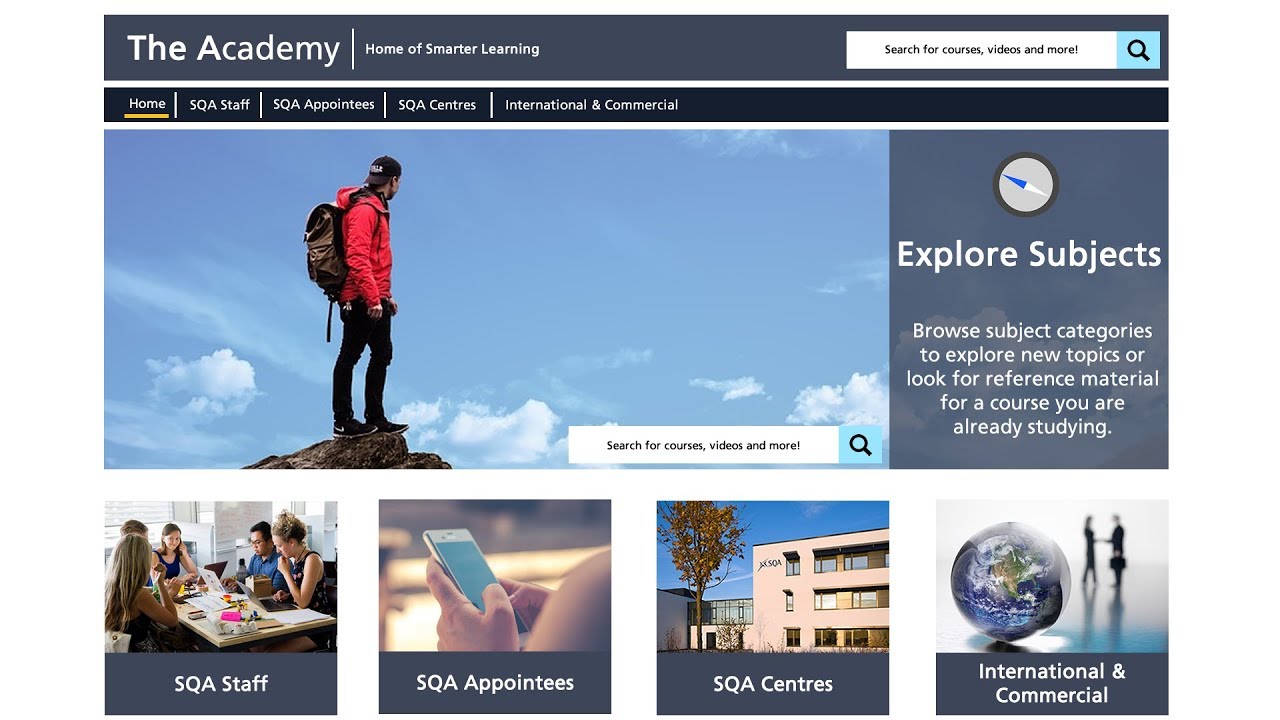**Detailed Caption:**

The webpage from "The Academy" features a prominent dark gray banner along the top. On the left side of this banner, "The Academy" is displayed in bold white text. To its right, separated by a vertical bar, the phrase "Home of Smarter Learning" is printed in smaller white text. At the far right of the banner is a white search bar.

Directly below the main banner, a slender black ribbon provides navigation options. From left to right, the options include Home, SQA Staff, SQA Appointees, SQA Centers, and International Commerce, with the Home option currently selected.

The webpage's main visual is a striking image of a hiker or backpacker standing on a mountain summit, perched on a small ledge with a steep drop-off. The scene is set against a backdrop of a blue sky scattered with fluffy white clouds. The hiker, a man, is dressed in a red jacket, black pants, and black shoes. He wears a black baseball cap with white text, turned backwards, and a dark brown backpack. At the bottom of this image, another search bar prompts visitors to "Search for Courses, Videos, and More."

To the right of this captivating image, on a dark gray background, white text invites users to "Explore Subjects." Below, a sentence encourages visitors to "Browse Subject Categories to Explore New Topics or Look for Reference Material for a Course You Are Already Studying." An adjacent graphic depicts a compass, consisting of a gray circle with a black border and a needle that is half white and half bright blue.

Further down, four squares showcase imagery related to the academy: people studying around a table, an individual using a smartphone, the exterior of a building, and a globe with two people shaking hands in the background.